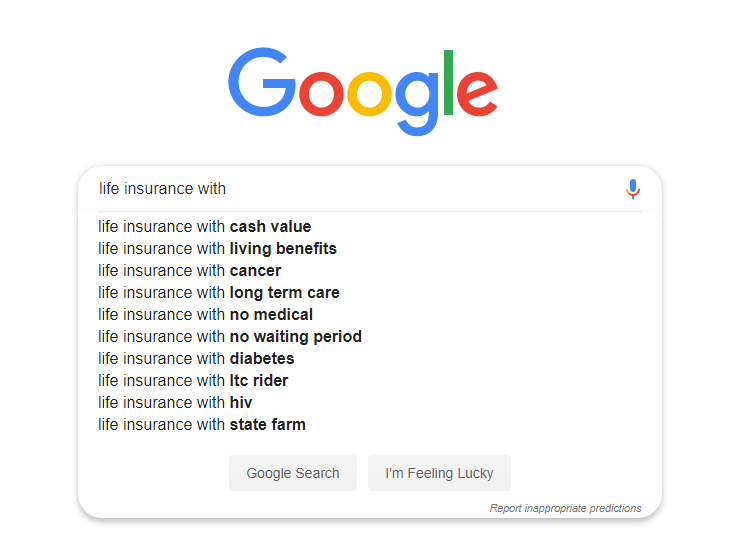The image displays a Google search interface prominently featuring the Google logo, which is rendered with its characteristic color scheme: blue 'G', red 'o', yellow 'o', blue 'g', green 'l', and red 'e'. Surrounding the search bar are various life insurance-related phrases such as "Life insurance with microphone," "Life insurance with cash value," "Life insurance with living benefits," "Life insurance with cancer coverage," "Life insurance with long-term care," "Life insurance with no medical exam," "Life insurance with no waiting period," "Life insurance for individuals with diabetes," "Life insurance with LTC rating," "Life insurance for those with HIV," and "Life insurance with State Farm." 

The search interface itself includes a gray "Google Search" button and another button that reads "I'm Feeling Lucky." Additionally, there is a note at the bottom right of the search box saying "Report inappropriate predictions." 

A subtle shadow effect can be observed around the edges of the search bar, and the text appears in 10 rows underneath the search functionalities. The overall design is clean and minimalistic, dominated by two prominent gray rectangular buttons: one for initiating the search and one for the "I'm Feeling Lucky" feature.